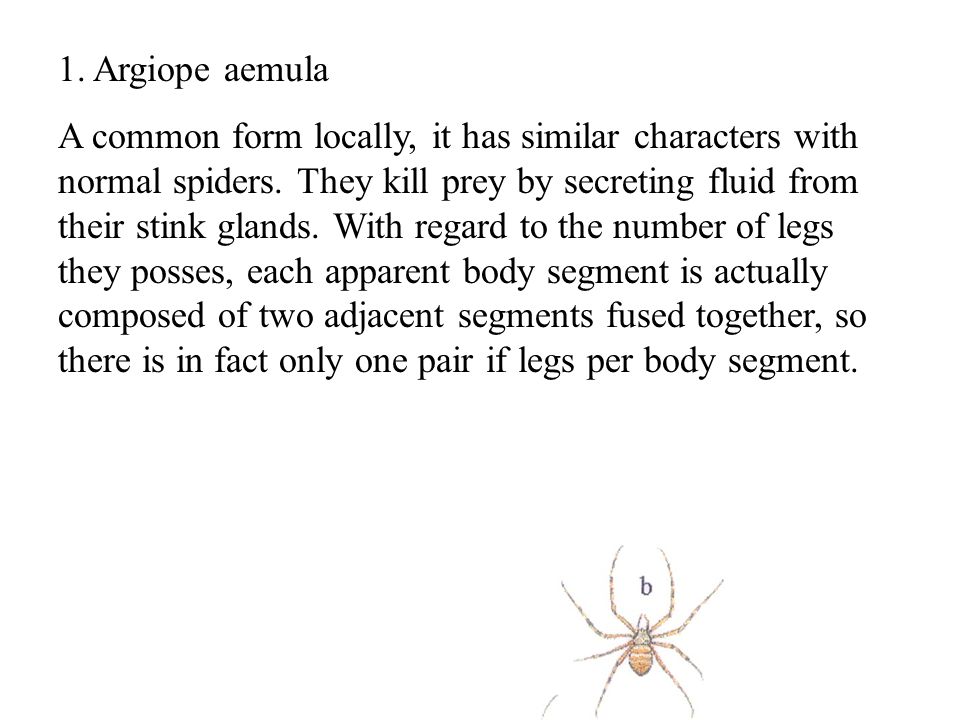This image resembles a page from an entomology book, featuring detailed text and an illustration. Dominating the top portion of the image, black typed text in an educational style describes a spider species, labeled "1. Argiope amula." The description highlights that it is a common local variety with characteristics akin to typical spiders. It details how these spiders kill prey by secreting fluid from their stink glands and explains that each apparent body segment is actually composed of two adjacent segments fused together, resulting in one pair of legs per segment. Despite a few textual typos, the information is clear. At the bottom right corner of the image, there is an illustration marked with a lowercase 'b' in Times New Roman font. The illustration depicts a brownish, gray-dotted spider with long, slender legs. The overall coloration of the image is monochromatic, with shades of black, white, and brown, ideal for a classroom or educational website.